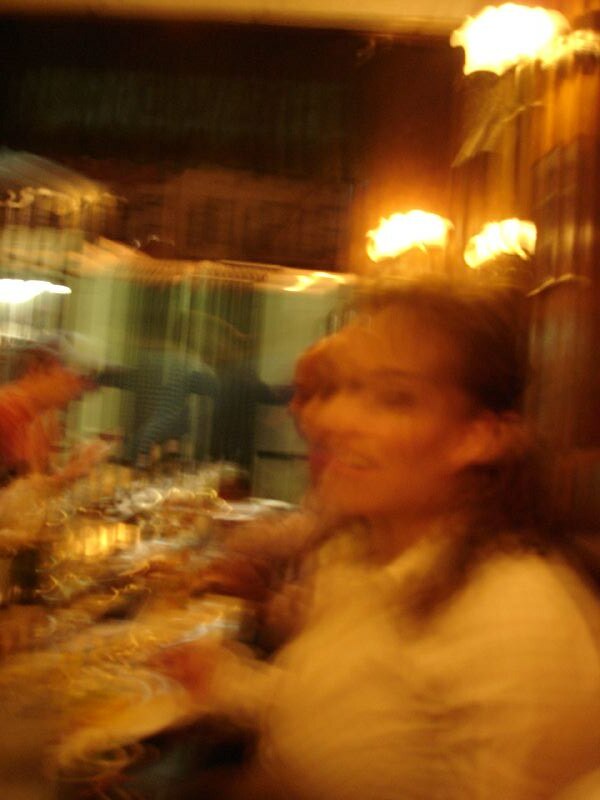This image captures a very out-of-focus and blurry dining scene, seemingly distorted by camera shake. Despite the blur, we can discern a cozy, possibly vintage European dining area, likely in a restaurant due to the high wall lamps. The centerpiece of the image features a young woman with dark brown hair, dressed in a white long-sleeved shirt. She is smiling and looking towards the camera, her right arm possibly holding a glass on the table adorned with glassware, placemats, and a centerpiece. Around her, other people are seated, engaged in conversation, though their features are indistinct due to the blur. The table is set with food and wine glasses, adding to the convivial atmosphere. The setting appears warm and inviting with soft, warm lighting and the ceiling in the background suggesting a low, cozy space.